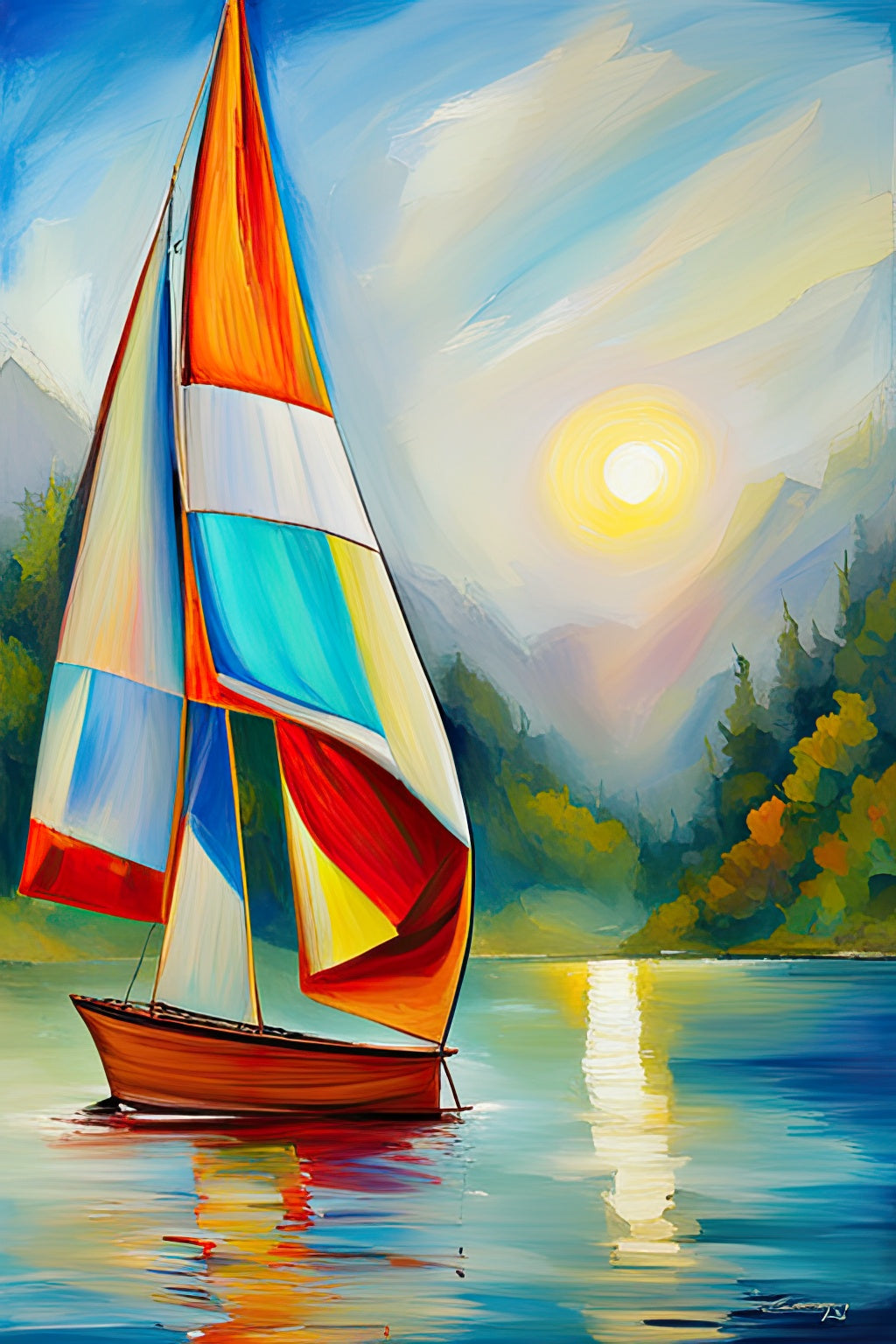This is a detailed oil painting, possibly created with both brushes and palette knives, rendered in portrait orientation. The main subject is a wooden sailboat with tall, striking multi-coloured sails that dominate the canvas. The sails exhibit a vibrant blend of hues including orange, yellow, red, blue, and white, arranged in a seemingly patchwork fashion that adds a dynamic element to the composition. The left sail features an intricate pattern of orange, yellow, red, and blue, while the right sail showcases sections of orange, white, blue, yellow, and a folded area with red, orange, and yellow shades.

The sailboat floats calmly on the water, which is mostly blue and mirrors both the boat and the sun that is positioned mid-sky, casting a warm reflection on the water's surface. The background reveals an evocative landscape with a lush bank of green trees interspersed with a touch of orange vegetation, transitioning into a serene valley that fades into distant mountains. The skies display a blue expanse dotted with fluffy white clouds, suggesting a clear, perhaps sunset-lit, atmosphere.

The painting features broad, expressive brushstrokes that infuse the scenery with a slightly abstract quality, foregoing detailed realism for a more emotive and implied depiction. These thick streaks are particularly noticeable in the sky, enhancing the textured, almost palpable visual experience. Overall, the piece is a vivid and richly textured portrayal of nature and tranquility.